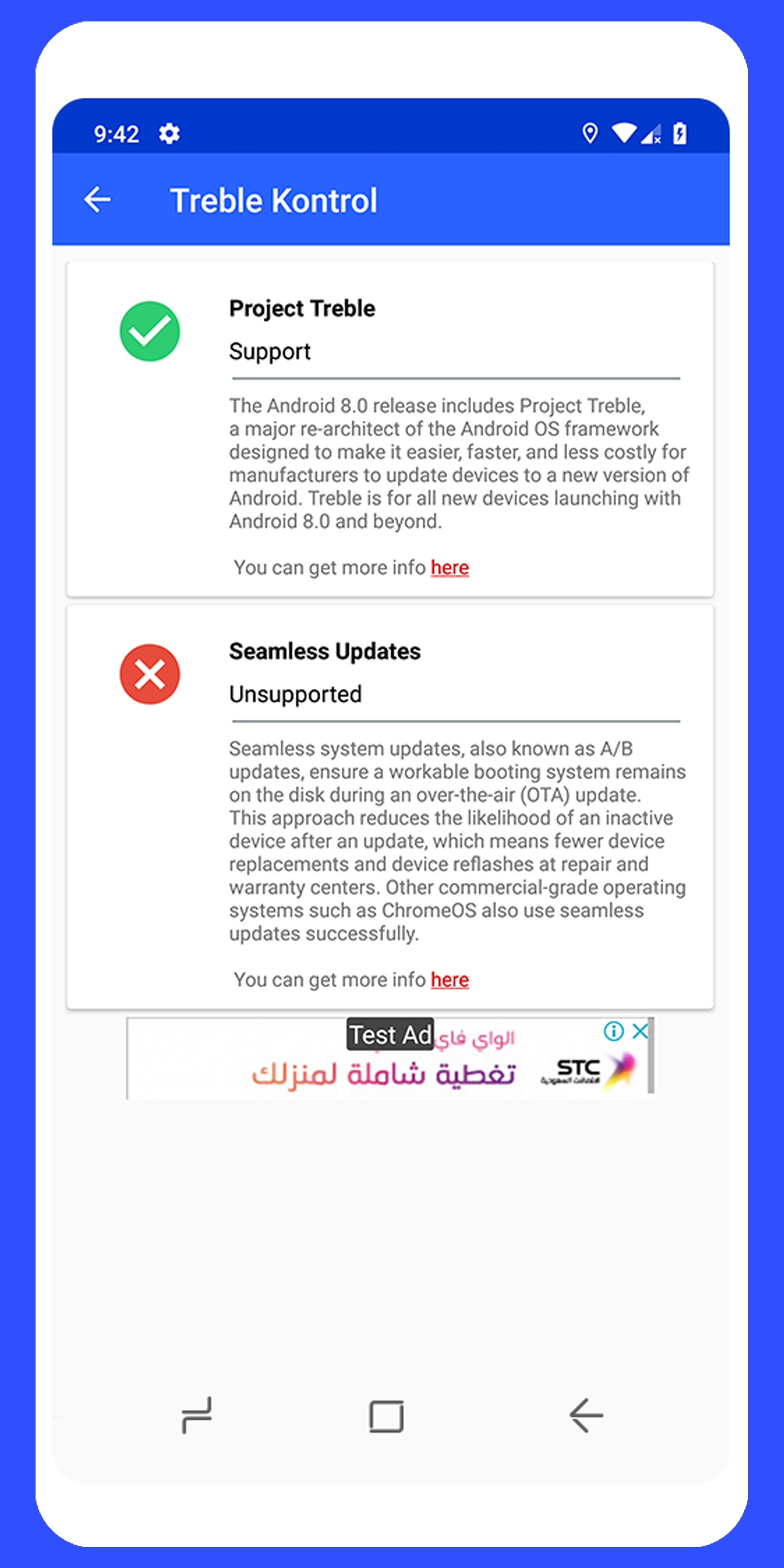The image features a message box with a white background and a medium blue border. At the top left corner, the number "942" is displayed. Just below this, there's a light blue section with an arrow pointing left, labeled "Treble Control."

Further down, a white area features a green circle with a white check mark and the text, "Project Treble Support." The caption beneath reads, "This Android 8.0 release includes Project Treble, a major re-architecture of the Android OS framework designed to make it easier, faster, and less costly for manufacturers to update devices to a new version of Android. Treble is for all new devices launched with Android 8.0 and beyond. You can get more info here."

Below this, another section features a red circle with an X mark and the text, "Seamless Updates Unsupported." The caption beneath explains, "Seamless System Update, also known as A/B updates, ensure a workable booting system remains on disk during an over-the-air update."